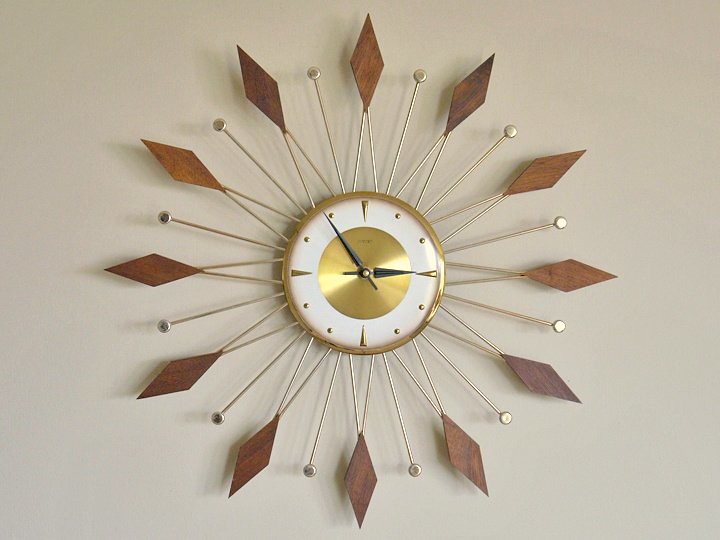This mid-century modern clock, mounted on a white wall, features an intricate and decorative design. The circular clock has a gold border and a gold center, with no traditional numbers on its face. Instead, the 12, 3, 6, and 9 positions are marked by large triangular indicators, while the remaining hours are marked by small gold circles. The black hour and minute hands point to a time of approximately 3:54. Surrounding the clock face is a distinctive pattern: alternating metal poles with small gold circles at their ends and pairs of metal poles coming together at wooden diamond shapes. The clock’s elaborate design casts shadows on the wall behind it, emphasizing its three-dimensional structure.